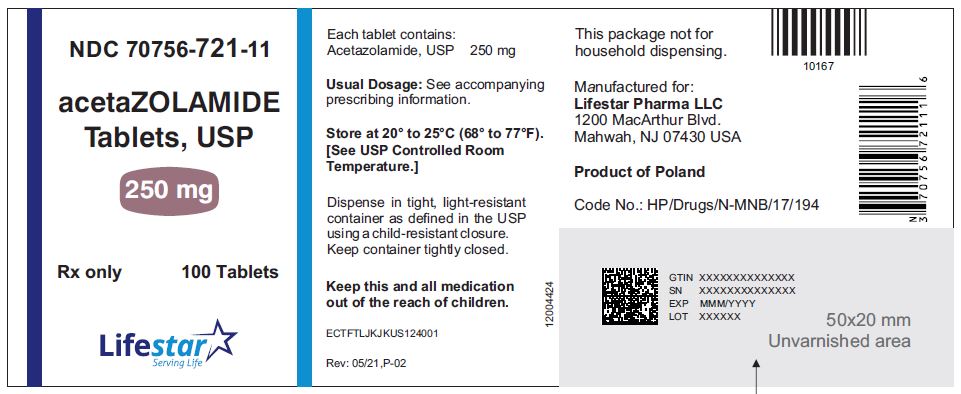This image features a detailed photograph of a prescription medication label. At the top, the label prominently displays "Acetazolamide Tablets USP" along with the dosage "250 milligrams." Positioned on the side, it indicates "RX only" and lists the quantity as "100 tablets." 

The midsection of the label is branded with the "Life Star" logo, complete with a star symbol and the motto "Serving Life." Further details in this area specify that "each tablet contains 250 milligrams" and advise the user to consult accompanying prescription information for the usual dosage instructions. There are also crucial storage instructions and a cautionary note to "keep this and all medications out of the reach of children." Additionally, it states that the package is "not for household dispensing."

The bottom section of the label informs that the medication is manufactured by Life Star Pharma LLC, located in New Jersey, and that it is a product of Poland. There is a code number and an ISBN code for scanning purposes, as well as another barcode at the top. The bottom right-hand corner features a gray rectangle containing additional scanning information, including a GTIN, SN, expiration date, and lot number. This area measures 50 by 20 millimeters and is unvarnished.